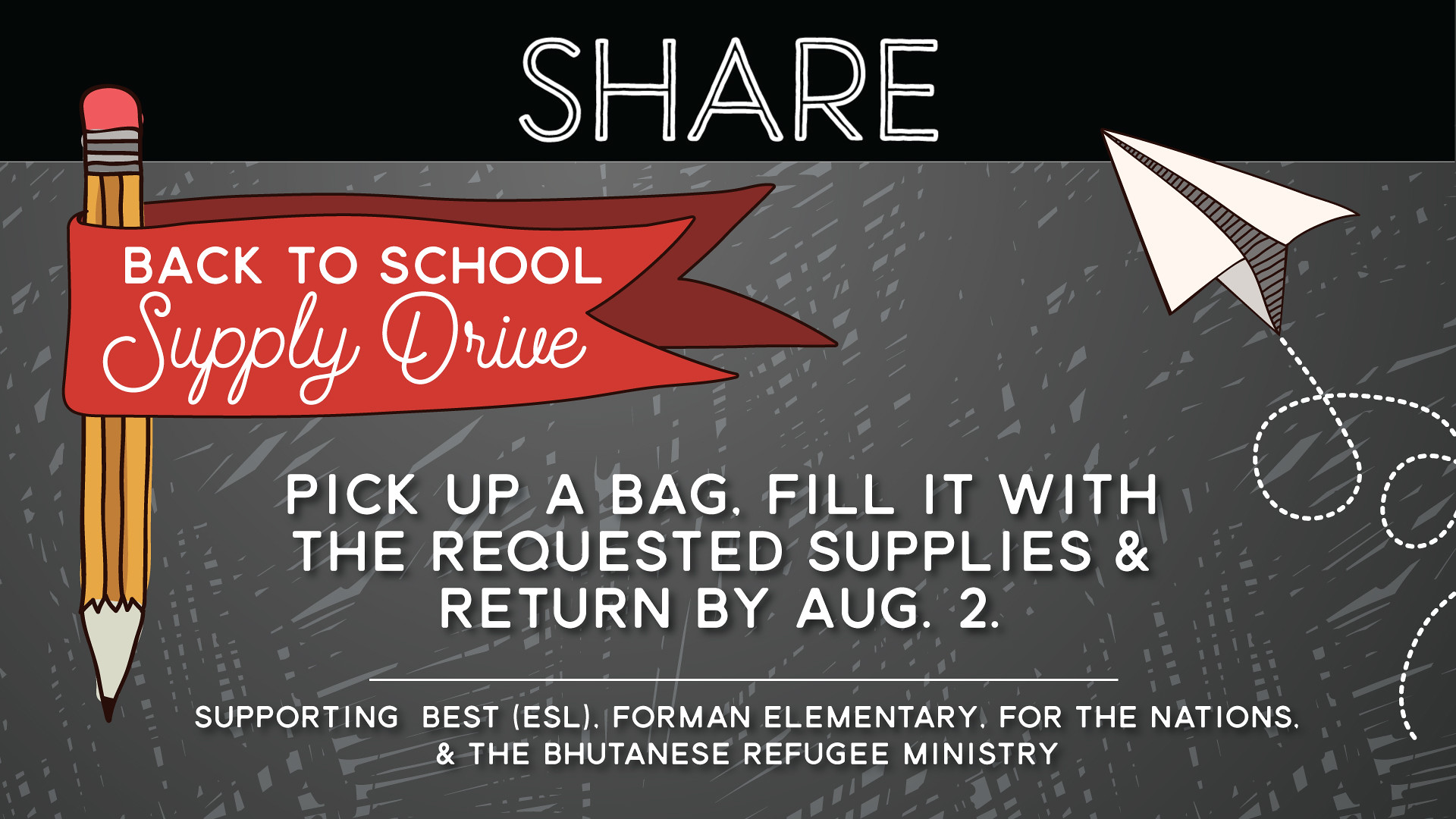This advertisement for a back-to-school supply drive prominently features a detailed drawing of a yellow pencil with an eraser at the tip, encircled by a red banner that reads "Back-to-School Supply Drive." At the top of the image, the word "SHARE" is clearly displayed in white text against a black background. To the right of the pencil, a paper airplane is shown flying, with whimsical curlicue lines trailing behind it. Central text instructs participants to "Pick up a bag, fill it with the requested supplies, and return by August 2nd." The background of this central text area is gray. At the bottom of the image, it notes that the initiative supports "Best ESL Foreman Elementary for the Nations and the Bhutanese Refugee Ministry."